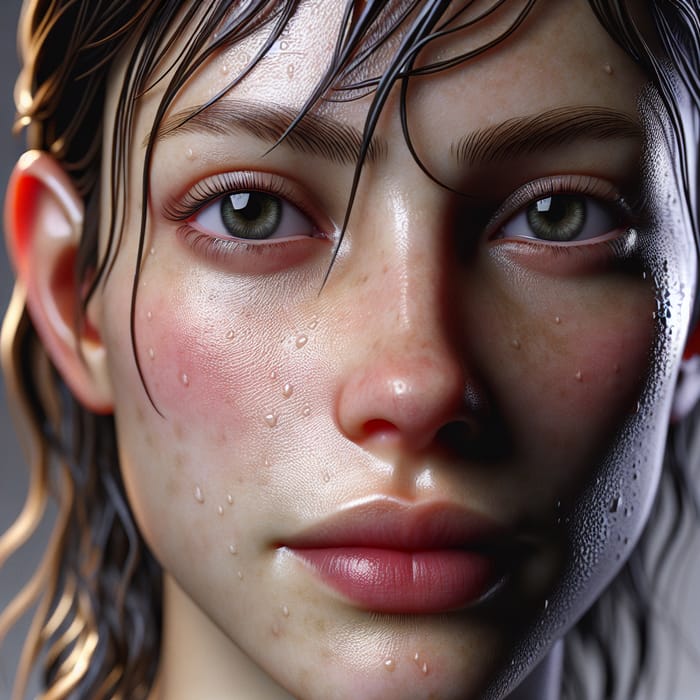The image depicts a hyper-realistic, digitally generated close-up of a woman's face. She has short brown hair, appearing wet, with some strands hanging down near her eyes, while the right side is tucked behind her ear. Her eyes are a striking green, and her expression is blank yet alert, accentuated by her wide-open eyes. Pink makeup adorns her face, which is scattered with fine, red freckles, especially around the nose. Her face and hair glisten with beads of sweat or water droplets. The right side of her face is brightly lit, contrasting with the darker left side. The image captures her from the middle of her forehead to her neck, highlighting these detailed features against a realistic but slightly artificial backdrop.